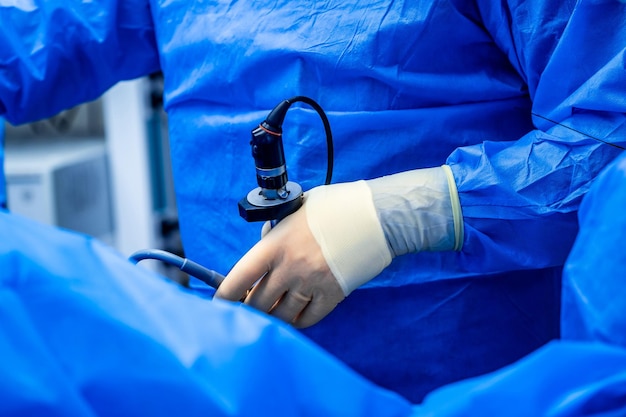The rectangular image, wider than it is tall, showcases an up-close view of a few individuals' torsos, primarily featuring blue, shiny, and waterproof outfits that resemble medical scrubs. These outfits might be surgical gowns, given their protective appearance. The focus is on the chest and arms, with one noticeable hand wearing translucent white gloves that extend over the wrist, revealing a gold ring on the ring finger. This hand holds an instrument with a black handle and a blue nozzle, which might also have a black cord and a tube. The background hints at a medical setting with glimpses of white storage cabinets and surgical equipment, completing the scene's clinical atmosphere. Another similarly dressed person is partially visible, reinforcing the medical context.